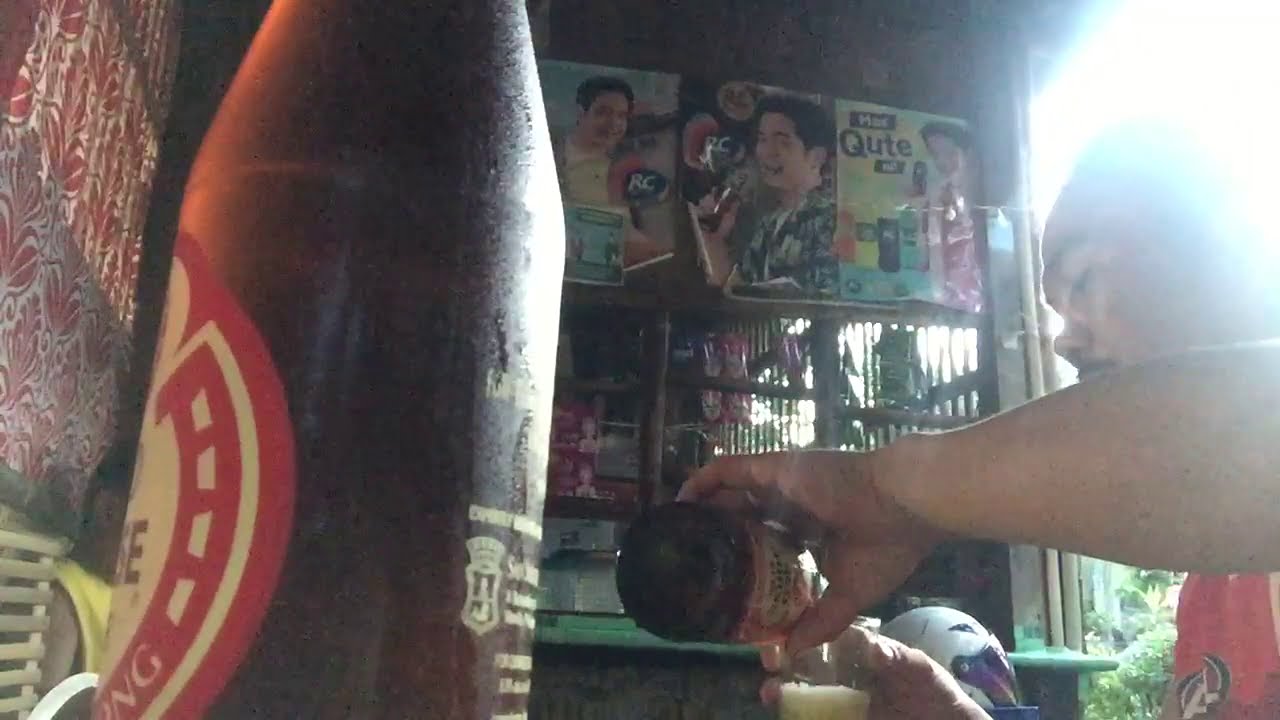This detailed photograph captures the intimate atmosphere of a small bar, likely in Southeast Asia, suggested by the subtle cultural elements present in the scene. In the bottom right of the frame, a man of possibly Filipino or Mexican descent, sporting a small black mustache and dressed in a red tank top or t-shirt, is seen pouring beer from a glass bottle into a nearly full glass. His side profile faces left, and he is backlit by sunlight filtering in from outside, highlighting the cozy, warm ambiance of the bar.

In the left foreground of the image, prominently, is a close-up of another beer bottle, displaying a red and yellow label, its details indistinguishable but indicative of an Asian or Pacific Islander brew. Behind the first man, the edge of another person is partially visible, adding to the sense of a communal, lively setting. The walls are adorned with posters featuring a man drinking beer, with lettering that includes Q-U-T-E, reinforcing the bar's casual and inviting vibe. Additionally, a motorcycle helmet rests on a bar stool in the background, hinting at the bar's roadside location. The entire scene evokes a laid-back, sunlit day, perfect for a refreshing drink among friends.